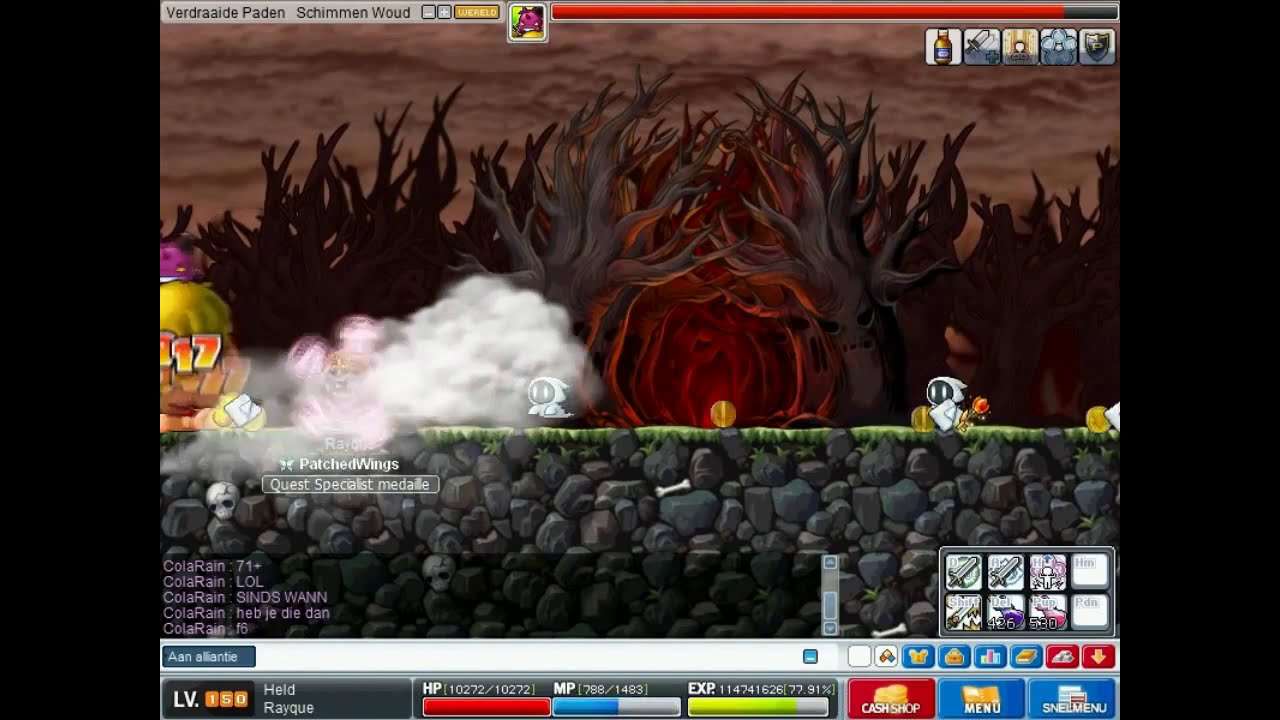The image is a detailed still shot from a video game featuring a dark, ominous forest scene. In the upper left corner, text in black font reads "Verta Side Paden Schimen Wood" along with a mostly filled red life bar. The sky is a dark brownish color, blanketed with thick clouds, which adds to the eerie atmosphere. The forest below shows numerous menacing trees with twisted, angry faces. These trees lack leaves and are various shades of gray, dark brown, and red, heightening the sense of dread. In the center of the image, two prominent trees with curved trunks form a glowing red hollow between them. A white cloud partially obscures the tree on the left.

The forest floor appears rocky with patches of stones, and several small bones and skulls are scattered about, enhancing the sinister environment. Positioned to the right is a small ghost-like character wearing a white hood, exposing a black face with large, glowing white eyes. Another similar ghost can be seen to the left center, partially obscured by smoke or clouds. Additional elements include a yellow object with indiscernible numbers and another purple creature, possibly a slug, partially visible on a structure to the far left.

Various game interface elements are also present: multiple icons labeled "HP," "MP," "EXP" with corresponding red, blue, and green bars, respectively, and other icons indicating "Cash Shop," "News," and "Menu." Additionally, there is a chat box at the bottom left displaying messages like "71+ LOL," presumably from a user named "Cola Rain." The bottom right corner holds more gameplay icons and stats, rounding out the detailed and atmospheric game scene.